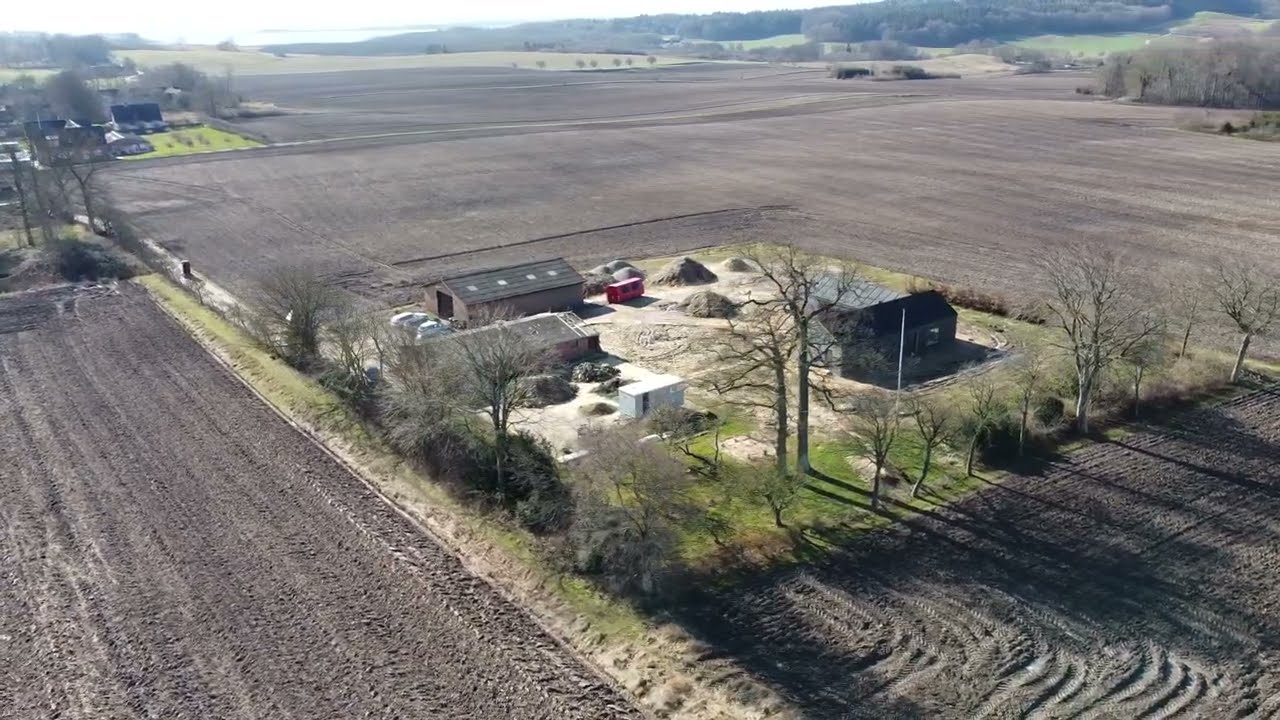This aerial shot captures a sprawling countryside dominated by large agricultural fields, segmented into various rectangular and square plots primarily composed of bare dirt and grass. The foreground features a vast expanse of freshly tilled brown dirt, marked by tire tracks from farm equipment. At the center of the image, enclosed by leafless trees and bushes, lies a farmstead with three large sheds, a storage trailer, and a red horse trailer behind one of the buildings. The farmstead also includes a couple of small white cars and a few outbuildings that likely serve as storage for agricultural tools. Extending from this central hub, more freshly tilled fields spread outwards. In the upper left corner, another plot contains a few homes, one white with a black roof, another brown, each surrounded by patches of green grass, suggesting these could be residences for farm workers or owners. The overall scene suggests late winter or early spring, with preparations for the planting season underway amidst leafless trees. In the distance, hay bales are visible across the fields, further emphasizing the agricultural nature of the landscape.